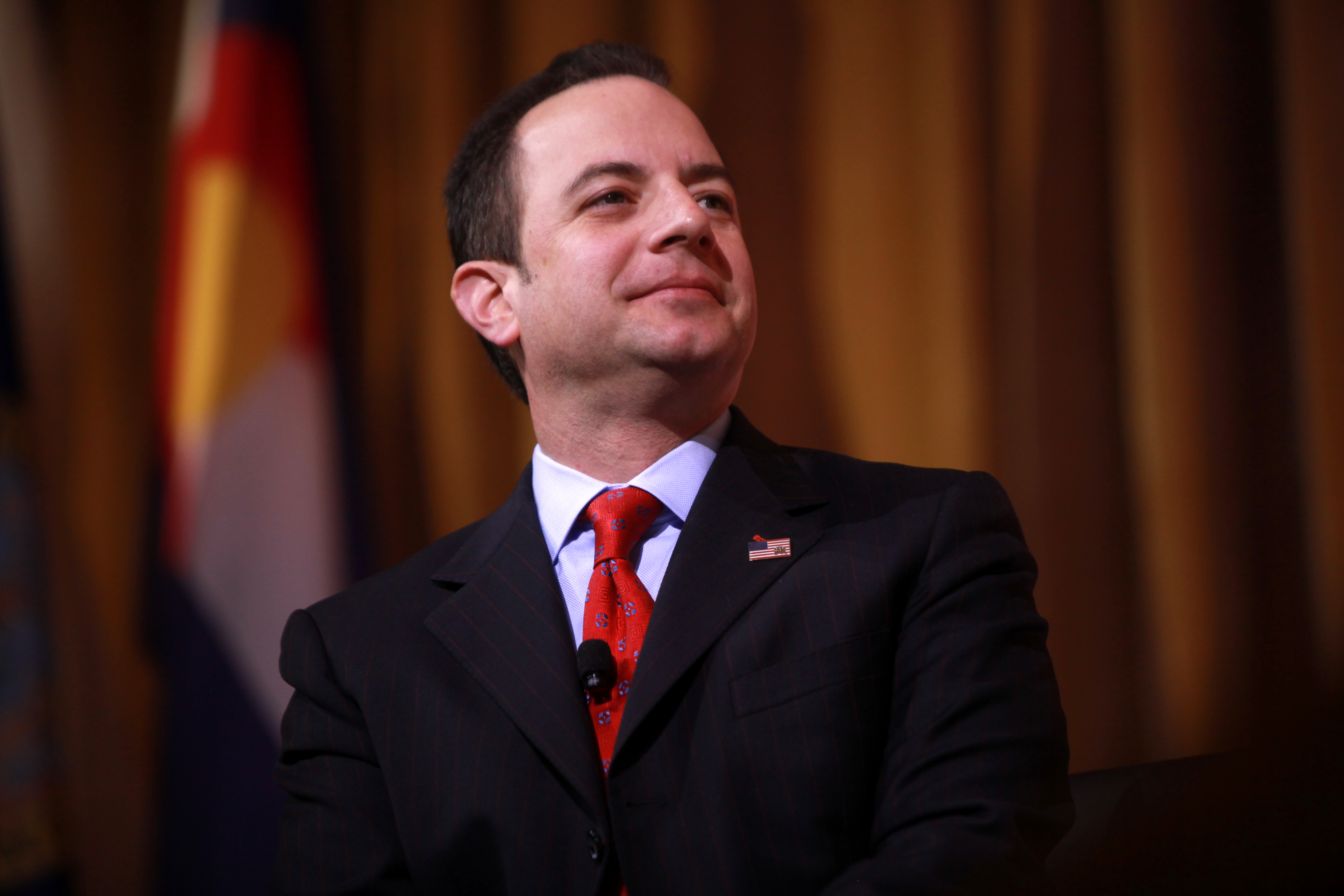A clean-shaven man with short dark hair and dark eyebrows is seated slightly to the left of center. His head is turned slightly to the left, and he is smiling. He is dressed in a black blazer and a white shirt, complemented by a red tie adorned with small designs. On his left lapel, he proudly wears an American flag pin that is red, white, and blue outlined in red. Behind him, a golden brown curtain serves as the backdrop, while to his left, a flag featuring the colors red, yellow, and white is visible. A microphone is discreetly attached to his tie, and he appears to be in a confident and composed stance.